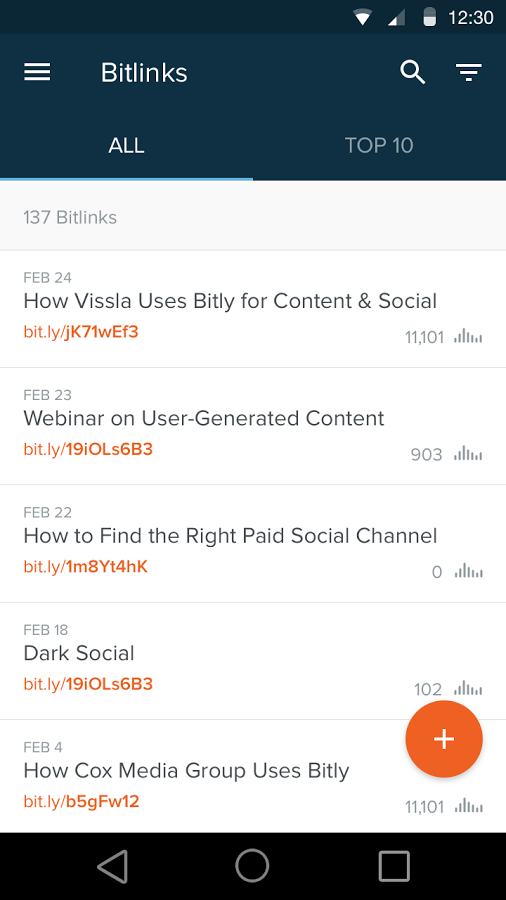The image is a smartphone screenshot featuring a web page header and URL list. The top smartphone header is black, displaying the time as 12:30 (unspecified AM or PM), a battery icon indicating about 50% charge, alongside Wi-Fi and wireless connection icons.

The web page header below is a midnight blue with "BitLynx" written in white on the left. BitLynx is a service that shortens URLs. Below the header, the options "All" and "Top 10" are visible against a white background. The page displays a list of 137 shortened URLs, each with a date, a headline, and a unique Bit.ly link.

Notable headlines include: 
- February 24th: "How Visla Uses Bitly for Content and Social"
- February 23rd: "Webinar on User-Generated Content"
- February 22nd: "How to Find the Right Paid Social Channel"
- February 18th: "Dark Social"
- February 4th: "How Cox Media Group Uses Bitly"

The font color for the headlines is light gray. At the bottom right, there's an orange circle with a white plus sign, and the phone's navigation bar is black with icons—a circle in the middle, a left-pointing triangle, and a square on the right.